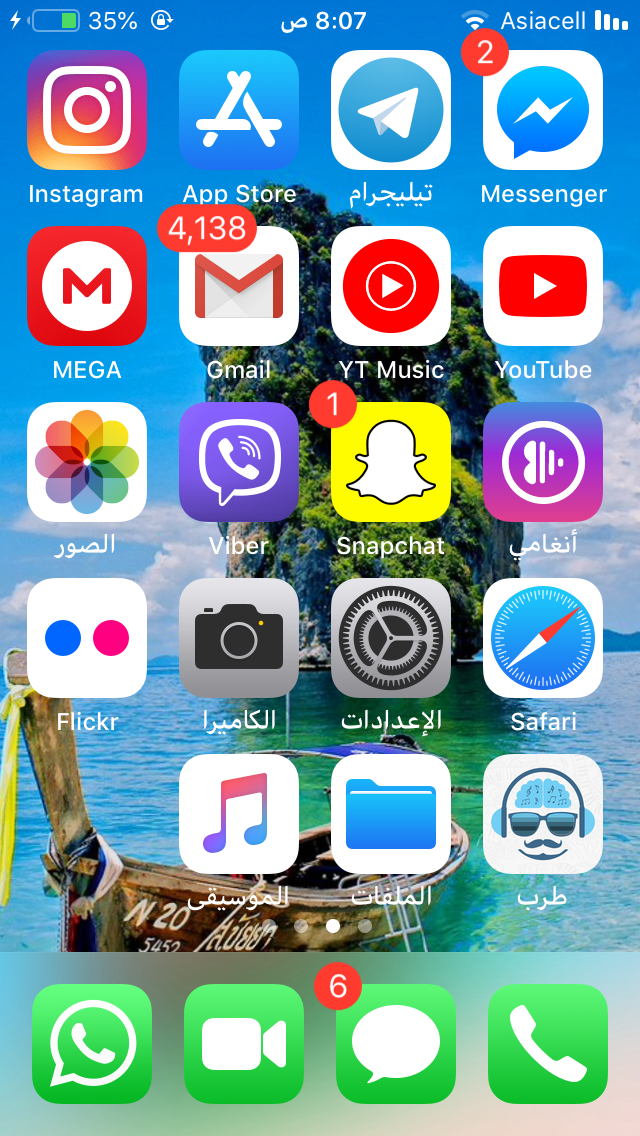This image is a screenshot taken on an iPhone displaying its home screen. The top right corner indicates the user is connected to the AsiaCell network, reflecting four bars of cellular service strength and two bars of Wi-Fi connectivity. The current time shown is 8:07, though it is unclear whether it is a.m. or p.m. The battery icon reveals that the phone is charging, with a green lightning symbol indicating an ongoing charge, and the battery level at 35%. Additionally, a lock icon suggests that the screen orientation is locked.

The home screen contains a total of 19 app icons, one of which is missing from its position. The visible apps include Instagram, the App Store, an app with a paper airplane icon, Facebook Messenger, YouTube, YouTube Music, Gmail, an app labeled Mega, Photos, Viber (similar to WhatsApp), Snapchat, a music-related app, Flickr, Camera, Settings, Safari browser, iTunes Music, a file folder app, and another music app. Along the bottom dock, there are icons for FaceTime, Camera, Messages (which shows 600 unread messages), and Phone.